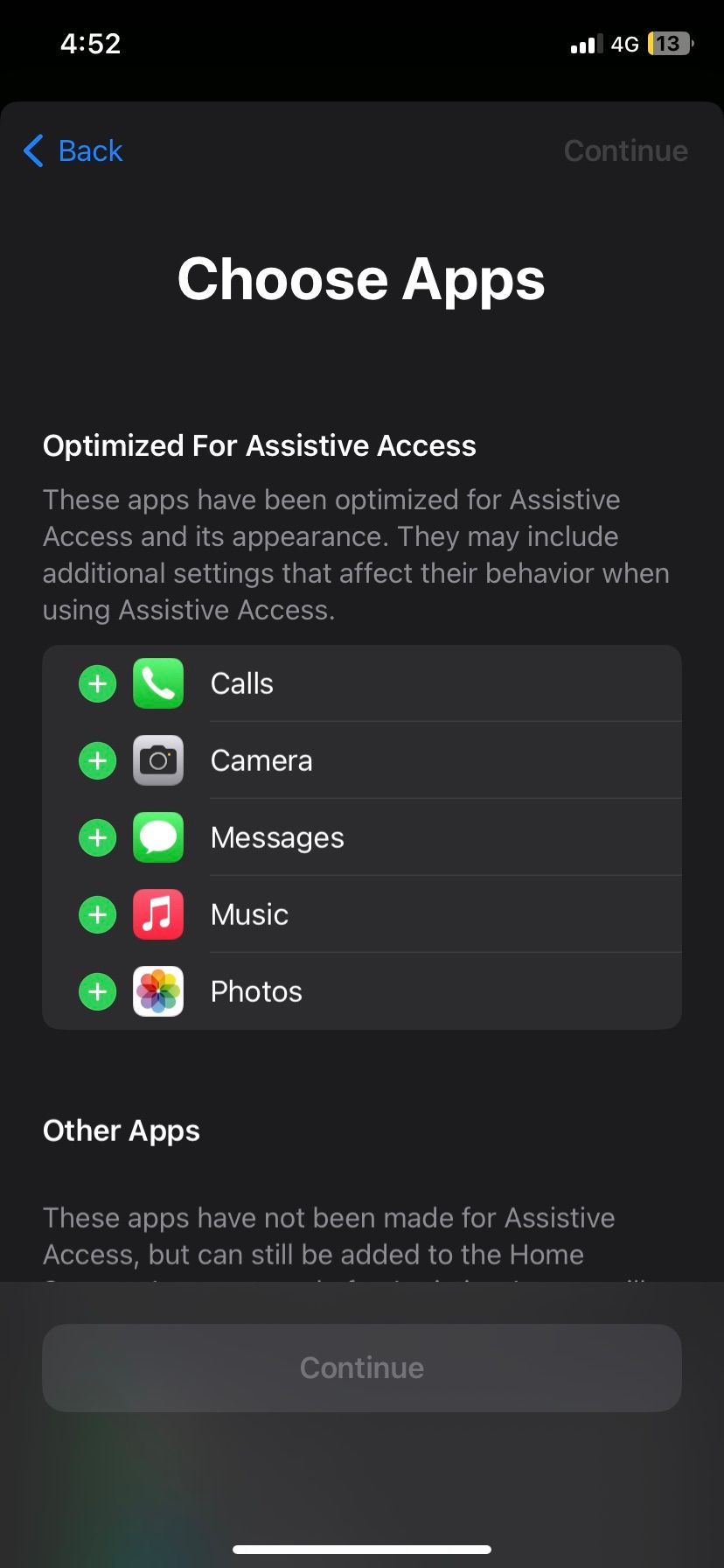The image is a screenshot taken from a phone's settings page shown in portrait orientation, appearing taller than it is wide. The background primarily features shades of black and gray accompanied by white text and various interactive boxes.

At the top of the screenshot, a horizontal black header displays the time "4:52" in white. To the right of the time, there is an icon indicating network connectivity with three out of four bars, a "4G" label, and a battery icon that is partly shaded yellow to denote 13% battery remaining.

Beneath this header, the background transitions to a gray shade. A blue back button is located on the left side, while a grayed-out "Continue" button sits on the right. Central to this section, a prominent header in white text reads "Choose apps," followed by a subheader "Optimize for Assistive Access." The accompanying description states, "These apps have been optimized for Assistive Access. They may include additional settings that affect their behavior when using Assistive Access."

Below this description, there are five elongated and narrow gray boxes, each representing different apps: Calls, Camera, Messages, Music, and Photos. Each app listing includes an icon and a green circle featuring a white plus sign.

Further below, the background turns darker, and in white font, it reads "Other Apps," followed by a brief description. At the very bottom of the screenshot, there is a semi-transparent border and another long, narrow "Continue" button, which is grayed out, indicating it is not currently clickable.